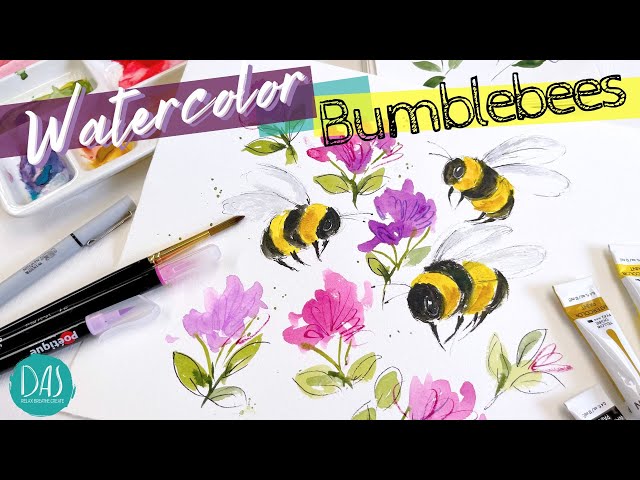The image is a photo of a watercolor painting, prominently featuring three bumblebees painted in black and yellow, flitting around purple and pink flowers, likely lavender and hot pink blooms. The painting is set against a white background. Overlaying the image, the title "Watercolor Bumblebees" is displayed. The word "Watercolor" appears in an elegant white script inside a translucent plum strip, while "Bumblebees" is in black bubble letters on a yellow background.

On the left side of the painting lie several tools used for its creation: a white paint tray with assorted paint colors (blue, green, yellow, red), a Sharpie, a thin watercolor brush, and a few markers, including a gray one and a shorter marker branded with "Poetique." Towards the bottom right corner of the image, there are three tubes of watercolor paint – identifiable colors include yellow, brownish bronze, and black.

On the bottom left of the image is a teal circle bearing the words "D.A.S., Relax, Breathe, Create." The background of the entire setup is framed by two black strips, one at the top and one at the bottom, with the central white painting area prominently displayed in between.